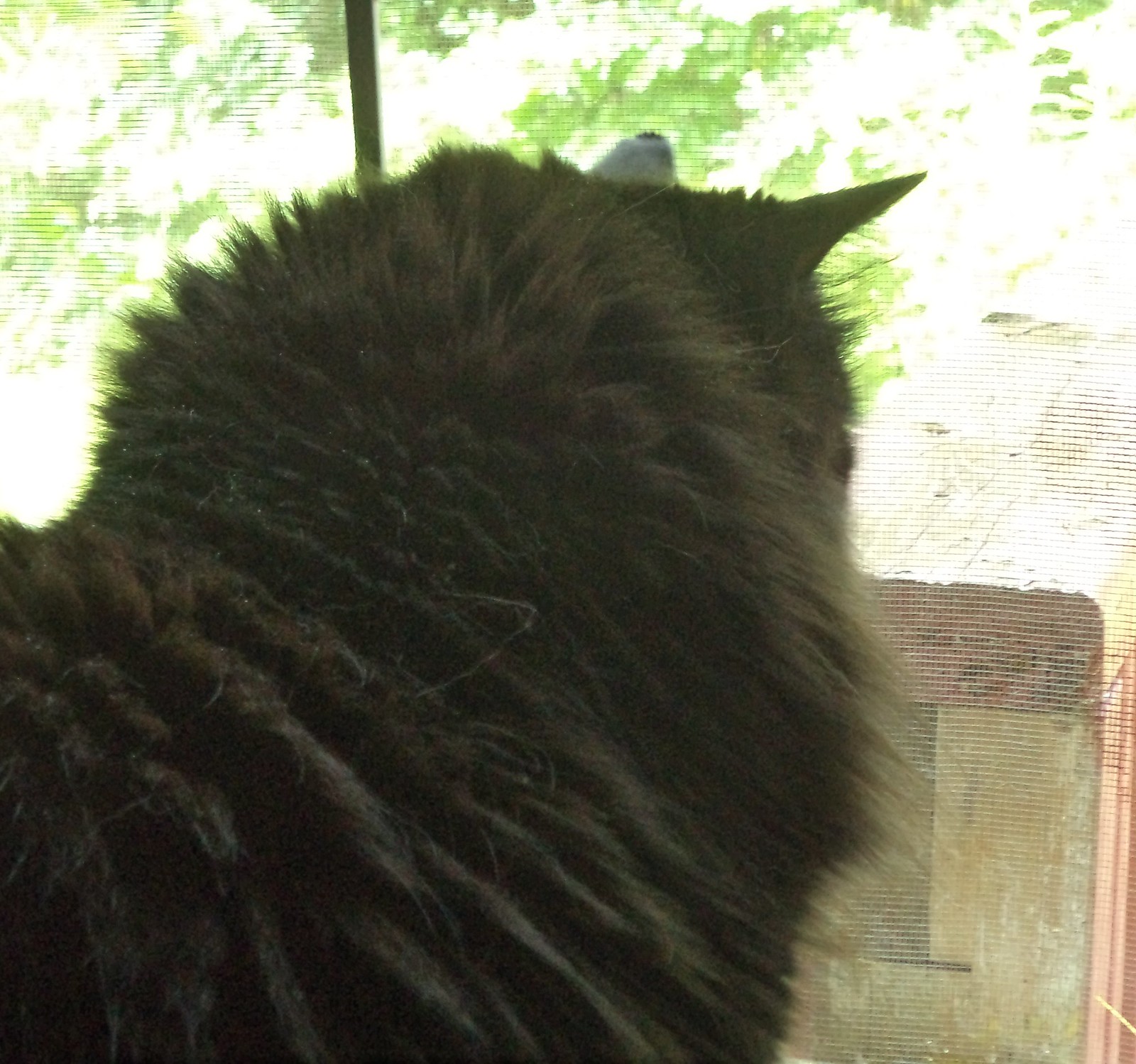The photograph captures the backside of a black cat, adorned with long, bushy fur with speckles of dandruff and stray strings. The cat's fur, primarily brown, appears fluffed up, indicating it is on edge. Perched at a screened second-story window, the cat's attention is fixed on something outside, possibly a bird. Although the face of the cat is not visible, an ear is discernible atop its head. The background reveals part of the roof of a neighboring building and some green leaves or trees, providing a natural backdrop to the scene.